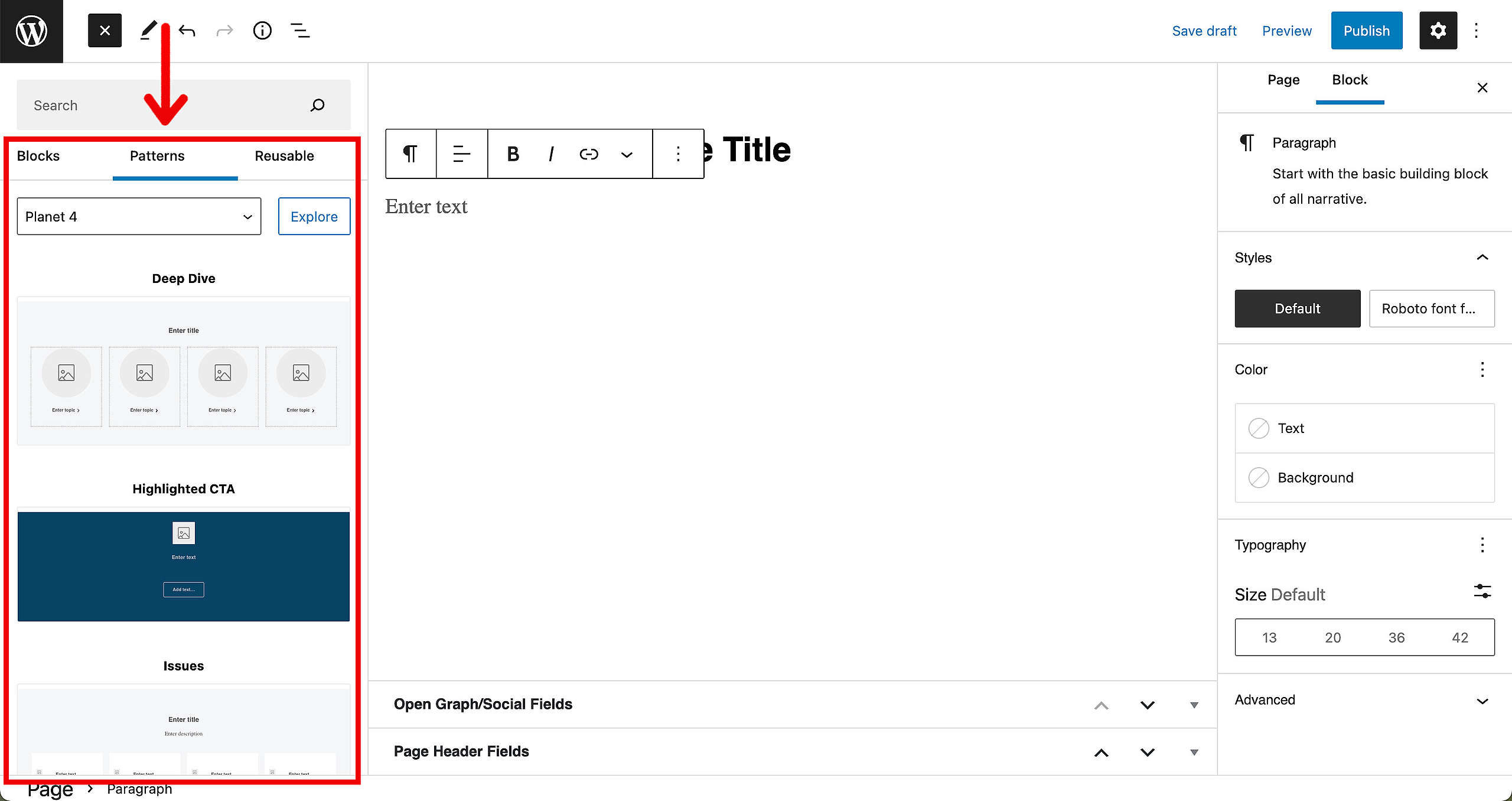This screenshot, taken from an unnamed website editing platform, captures a detailed view of the editing interface. In the top-left corner, there's a distinctive black box featuring a white "W" within a white outline circle, likely representing the website's logo. Adjacent to it, there's a smaller black box housing a white "X," typically used for closing the window or exiting the screen. 

Next to these elements, there’s a set of editing tools which include a pen icon with an underline, indicating that the pen tool is currently selected. Alongside it, two arrows pointing left and right represent the undo and redo functions. Further to the right, icons for additional options are displayed: an "I" in a black outline circle, and three horizontal lines arranged in a stair-step formation.

To the far right, in the top row, are the save and publishing options. The words "Save Draft" and "Preview" appear in blue font, followed by a blue box with the word "Publish" in white font. A black box containing a cogwheel icon indicates the settings menu, and next to it, three vertically stacked dots suggest more options.

On the left-hand side of the interface, beneath a search box, are three categories labeled "Blocks," "Patterns," and "Reusable," indicating different sections of the project. The central area shows the editable project surrounded by a red box, with an arrow pointing downward at it, suggesting a focal point for the user. In the middle of the screen, the project content is displayed and is ready for editing.

To the right, further customizable settings appear, categorized under "Page" and "Block". These options include sub-settings for "Paragraph," "Styles," "Color," "Typography," "Size," and "Advanced Options." At the bottom center of the screen, additional options labeled "Open Graph or Social Fields" and "Page Header Fields" are also visible, likely linked to metadata and header configurations. This comprehensive interface layout indicates an active engagement in a detailed web editing project.